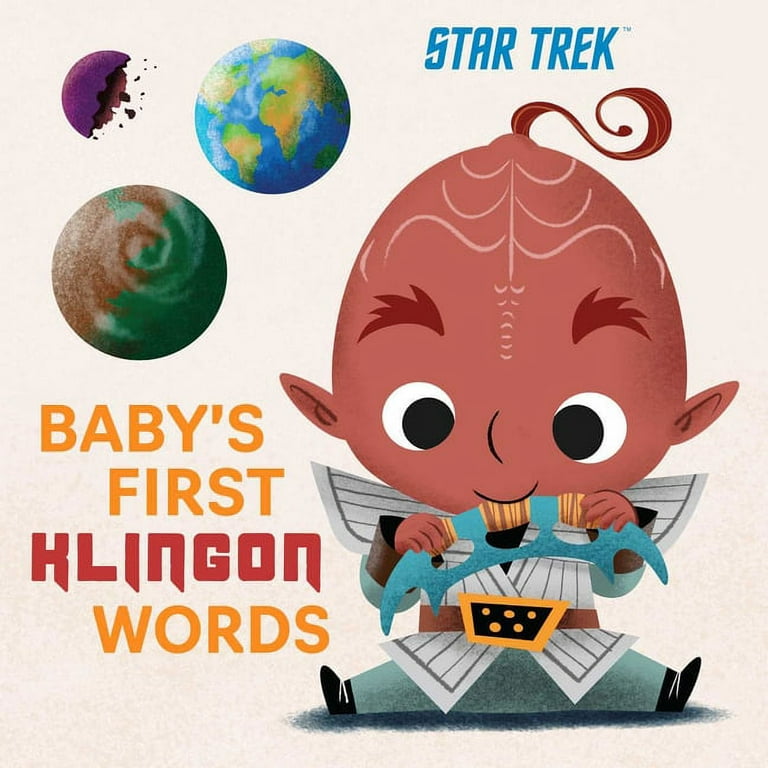The image is a cartoon-style drawing of a young Klingon baby from the Star Trek series. The baby, characterized by his mountainous ridges on his head and pointy ears, sits in the bottom right corner of the image. He has a prominent curl of hair on top of his head, bushy eyebrows, and medium brown skin. His outfit consists of a white and gray striped shirt, a stiff pointy collar, a brown belt with an orange and brown buckle, blue-gray pants, and little black shoes. He holds a blue spiky Klingon warrior tool in his mouth. 

In the background on the top left, there are three planets: Earth, a unique green and orange planet, and a half-planet resembling an eggshell or a chewed-up cookie. The background is gray, creating a stark contrast to the colorful elements. The caption "Baby's First Klingon Words" is at the bottom left, while the word "Star Trek" is prominently displayed at the top right. The baby is looking straight at the viewer, with black and white eyes focused centrally, giving a cute yet fierce expression fitting for a young Klingon.